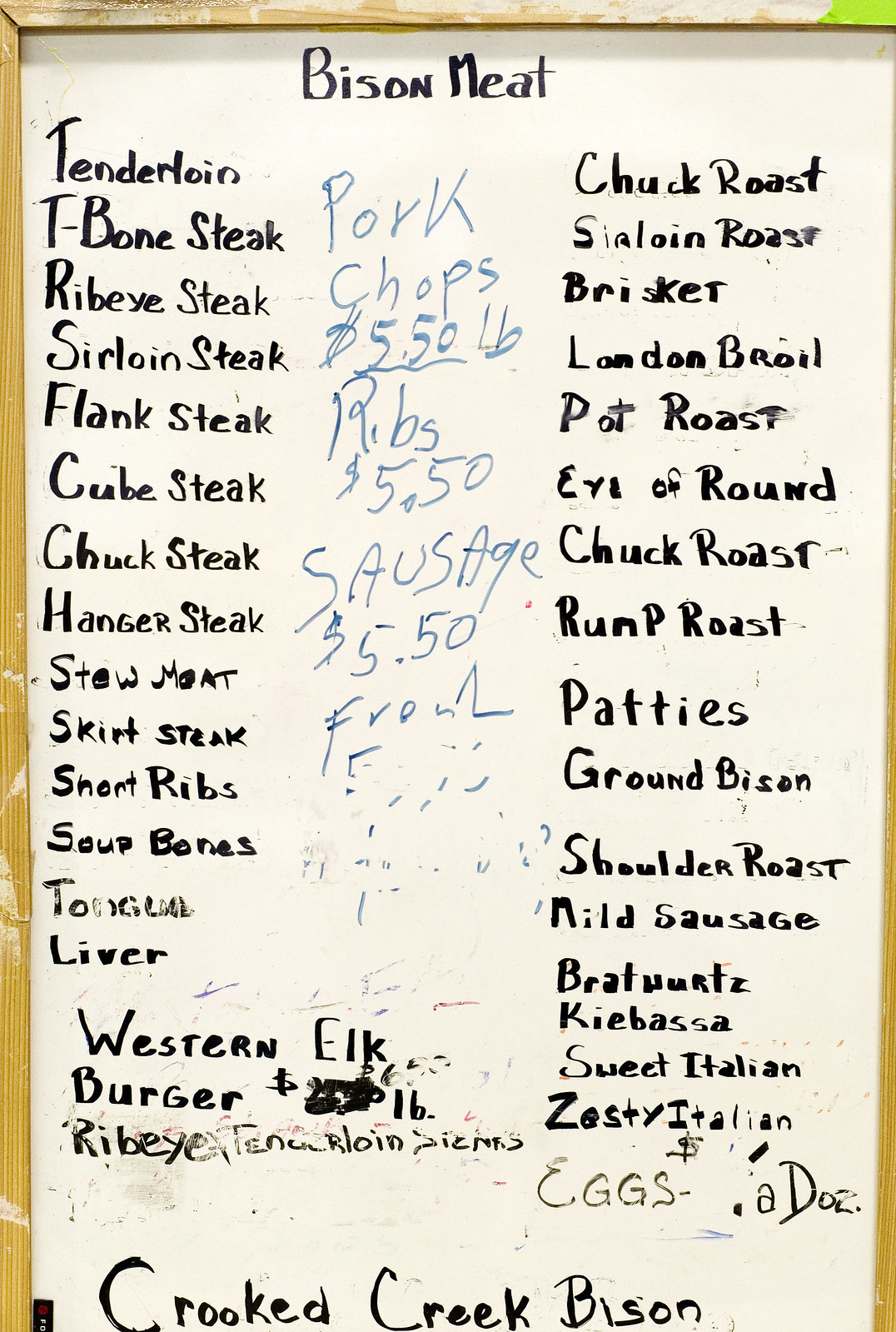The image captures a whiteboard menu featuring a variety of meat products. At the top, "Bison Meat" is prominently written. On the left-hand side, a comprehensive list includes: tenderloin, T-bone steak, ribeye steak, sirloin steak, flank steak, cube steak, chuck steak, hanger steak, stew meat, skirt steak, short ribs, soup bones, tongue, liver, and Western elk burger. Notably, the price for the Western elk burger has been scribbled out. Additionally, the words "ribeye" and "tenderloin steaks" are partially crossed out at the end.

On the right-hand side, another list includes: chuck roast, sirloin roast, brisket, London broil, pot roast, eye of round, chuck roast (listed again), rump roast, patties, ground bison, shoulder roast, mild sausage, bratwurst, bratwürst, kielbasa, sweet Italian, zesty Italian, and eggs (with the price per dozen also scribbled out).

Running down the middle of the board, written in blue marker, is a partially erased list. The legible items are: pork chops for $5.50 per pound, ribs for $5.50, and sausage for $5.50. The remainder of the list has been erased.

At the very bottom of the whiteboard, "Cooked Creek Bison" is written, finalizing the collection of offerings.